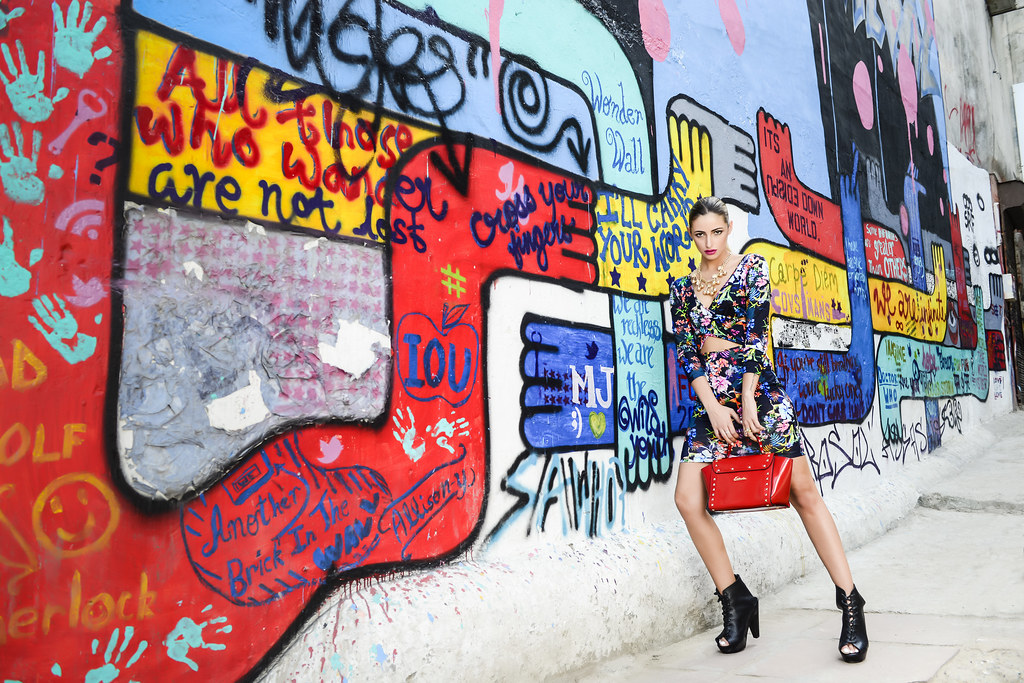In this vibrant street-style photo, a model is striking a poised stance against a vividly graffitied wall, adorned with a mix of bold red, yellow, blue, white, and pink hues, alongside various written captions like "I owe you," "cross your fingers," and "all those who wander are not lost." Dressed in a chic, floral two-piece ensemble featuring a cropped top with a low V-neck and three-quarter length sleeves, paired with a mini skirt, she puts forward a confident and edgy look. Her slicked-back hair and eye-catching red lipstick accentuate her striking facial features. She accessorizes with a necklace and a pair of black high-heeled peep-toe booties that lace or buckle up the front. In her hands, she elegantly holds a red oblong handbag with a single handle and rivet detailing, likely the focal product of the shoot. The setting is a regular city sidewalk, adding an authentic urban vibe to the overall composition.